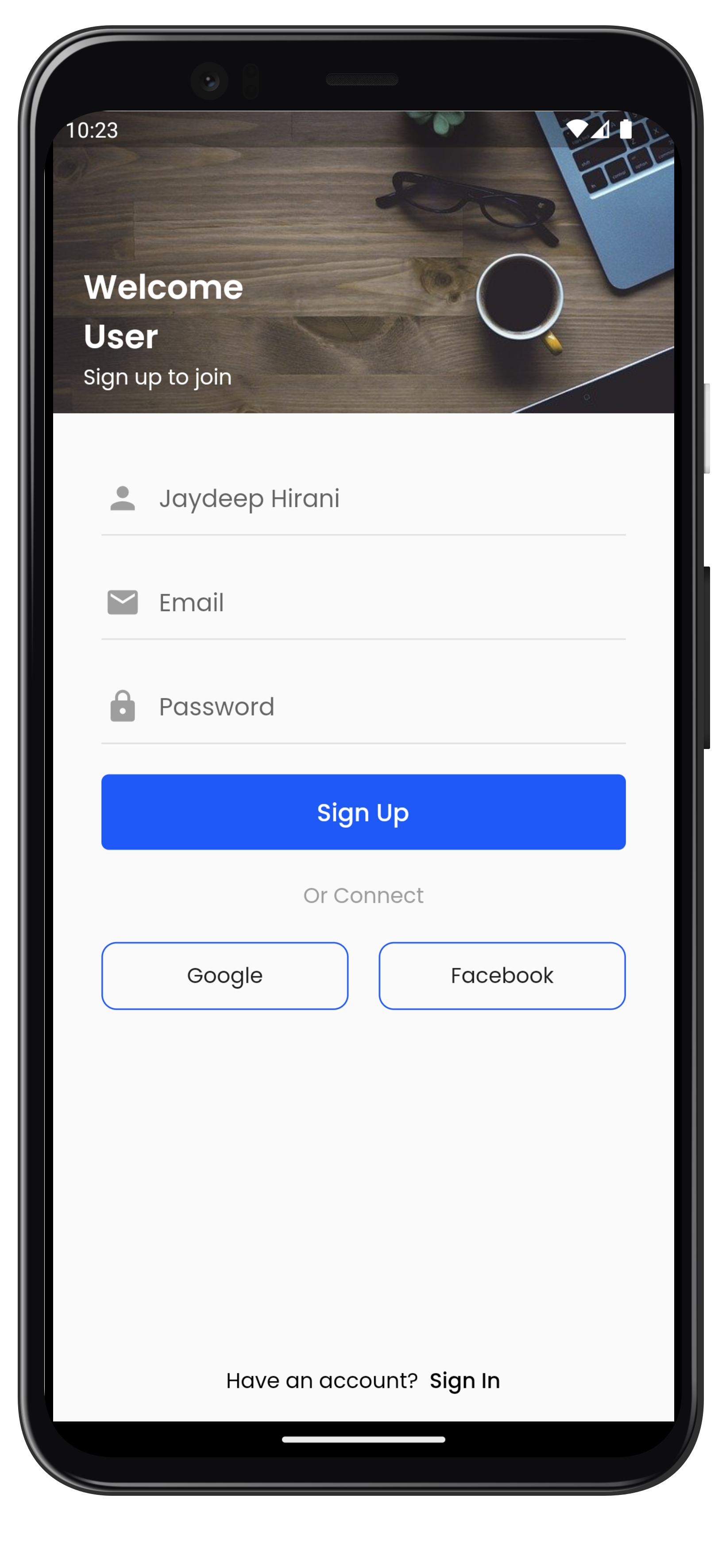This image features a cell phone showcasing its physical casing. On the right-hand side of the device, there are several buttons. The screen displays the time as 10:23, positioned in the upper left corner. The phone is currently on a log-in page. At the top of this page, there is an image depicting a top-down view of a table. The image includes a laptop keyboard and a coffee mug on the right, and a pair of glasses. In the bottom left of this picture, the text reads "Welcome User, sign up to join." Beneath the image, there are input fields for an email address and password.